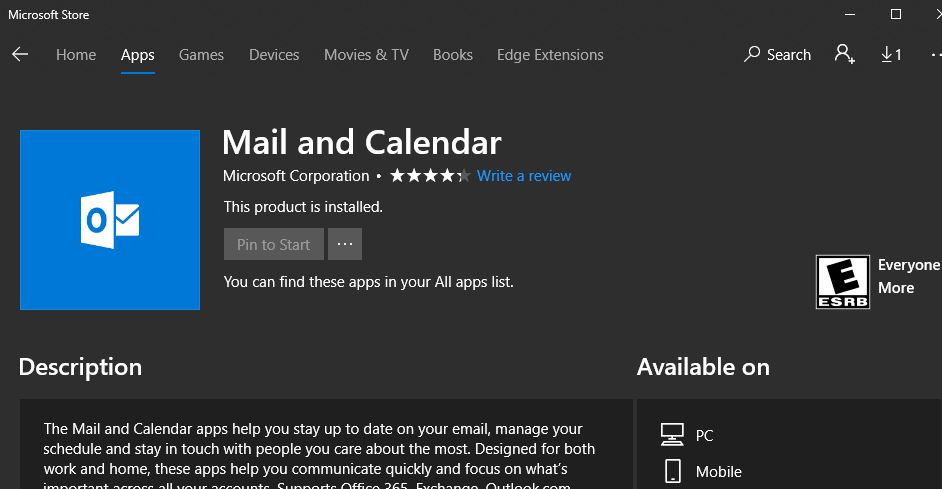A screenshot of the Microsoft Store is displayed with the focus on the Mail and Calendar app. The store interface has a black background with sections labeled as Home, Apps, Games, Devices, Movies & TV, Books, and Edge Extensions written in white text. The "Apps" section is selected, indicated by a blue underline and bold text.

Directly below, the Mail and Calendar app is showcased. It is rated 4.5 out of 5 stars and developed by Microsoft Corporation, with the status showing it is installed on the device. An accompanying icon features a blue background with a white envelope outlined in blue and a white square containing a blue circle.

Options such as "Pin to Start" are available, and users are informed that the app can be found in their All Apps list. On the right-hand side, an "Everyone" rating signifies that the app is suitable for all ages. Additionally, the app is noted to be compatible with both PC and mobile devices, depicted by computer and phone icons.

The app's description reads: "The Mail and Calendar apps help you stay up to date on your email, manage your schedule, and stay in touch with people you care about the most. Designed for both work and home, these apps help you communicate quickly and focus on what's important across all your accounts." It also highlights support for Office 365 and Exchange for Outlook.com, emphasizing its robust functionality for both personal and professional use.